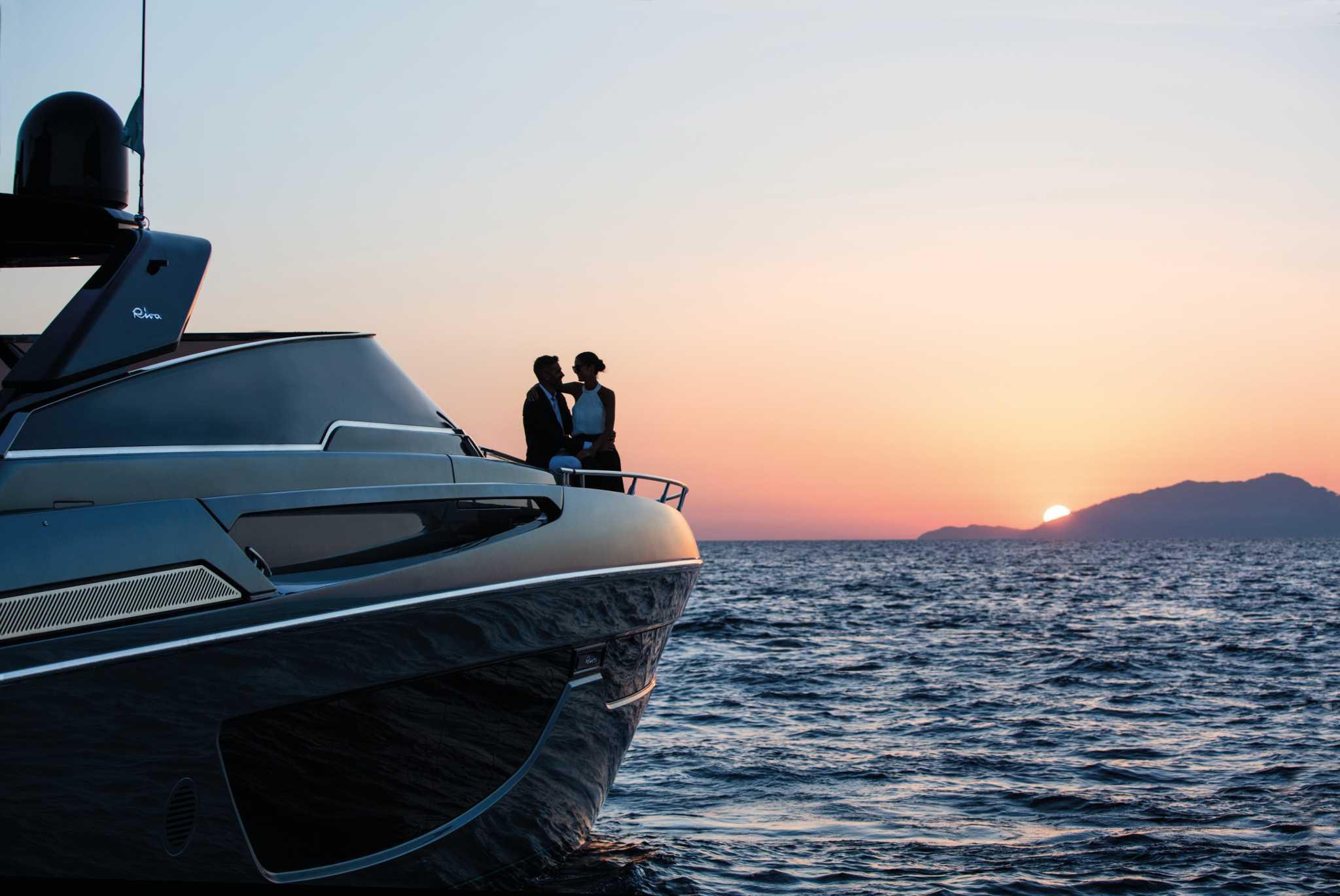The photo captures an intimate moment on a sleek, modern black yacht, named Riva, gliding on the calm, rippling ocean during sunset. The sky is a soft gradient of pastel blue, orange, pink, yellow, and purple as the sun sets over a mountain on the right of the image, casting a warm, romantic light. On the deck of the boat, towards the left side, a couple is seated on the bow. The man, dressed in a black suit with a white shirt and striped tie, sits close to a woman wearing a white halter top and black skirt, her hair elegantly styled in a bun. They are face to face, embracing lovingly, with the woman's arm around the man's shoulder, sharing an intimate and joyful moment amidst the serene natural beauty.